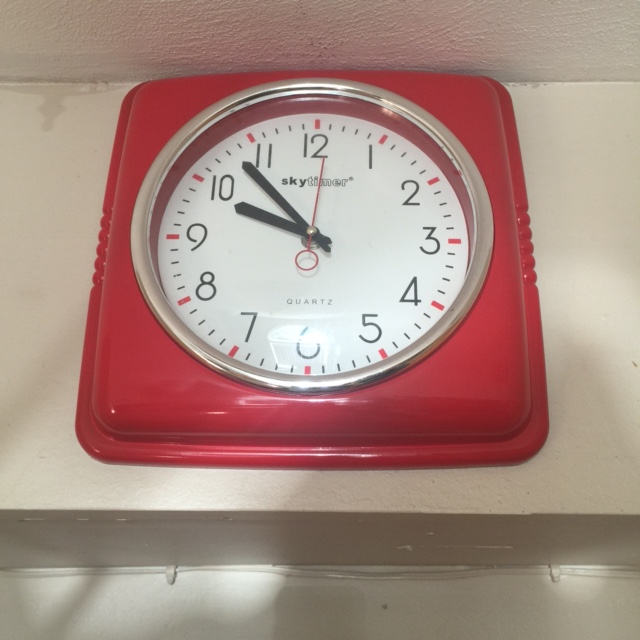This detailed photograph captures a square, retro-styled red clock prominently mounted on a pristine white wall. The white wall extends from the top edge of the image, with a subtle glimpse of the white ceiling visible. The clock face, encased in a sleek silver rim, features a white background accented by a combination of black and red dashed lines. The clock's hands include two black and one red, all pointing towards black numerals. The silver trim reflects a flash of light, adding a touch of brilliance to the retro aesthetic. Shadows cast underneath the clock enhance the depth and dimension of the image. Notably, there is visible water damage towards the top of the wall, contrasting with the spotless section of the backdrop. The photograph’s high quality and clarity emphasize these intricate details, making for an engaging and visually compelling image.